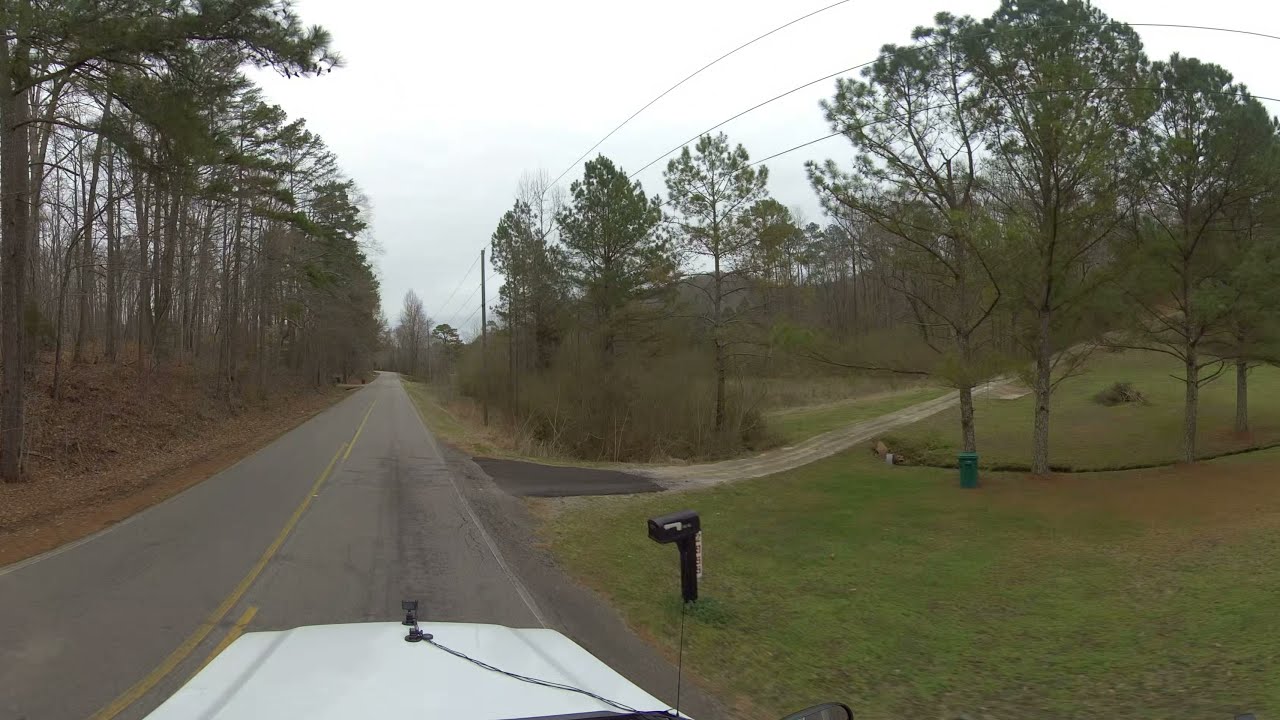The image depicts a rural, two-lane roadway, captured from a vehicle, likely a truck, traveling down the street. The road, composed of black-gray asphalt and marked by a yellow double line, is surrounded by a countryside landscape. On the left side of the road, the ground rises slightly, covered in brown earth and scattered leaves, with a mixed forest of bare deciduous trees and green evergreen trees in the background. On the right side, there is a well-maintained lawn with short, freshly cut grass. A large, black residential mailbox stands prominently in the foreground, indicating the entrance to a residential driveway. The driveway, made of brown dirt, winds up the grassy area towards a house, and next to it lies a green dumpster. Power lines run alongside the road, receding into the distance. The scene has a gray, wintry feel, with many trees devoid of leaves, further emphasizing the rural and tranquil setting.